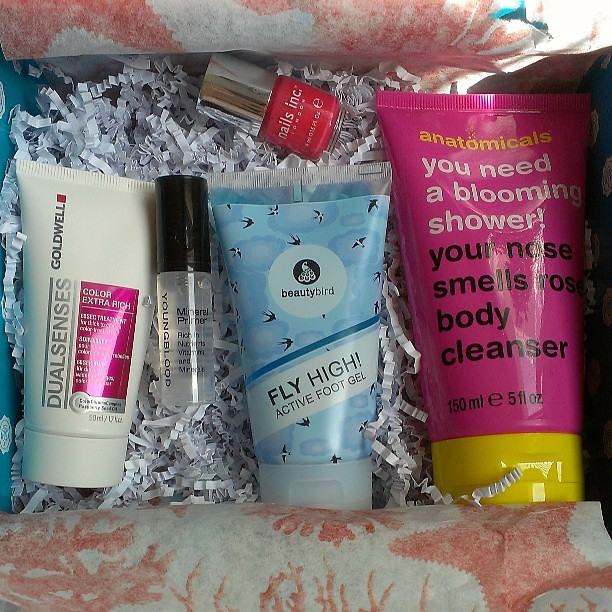The image depicts an open gift box lined with light pink star-patterned tissue paper and cushioned with crimped white paper strands. Inside the box are five distinct beauty products. On the left, there is a white tube labeled "Goldwell" with a small red box above it, and "Dual Senses" written sideways within a gray vertical bar. This tube contains color extra rich care for hair. Next to it is a transparent cylindrical bottle with a black cap, labeled "Youngblood Mineral Primer." In the center of the box, a blue tube features a circular logo with a bird symbol and is branded "Beauty Bird." It also has illustrations of blue birds in flight and is labeled "Fly High Active Foot Gel" in diagonal text. To the right, the largest item is a pinkish-purple tube with a yellow cap, labeled "anatomicals" in yellow text, followed by "You need a blooming shower," and "your nose smells of rose body cleanser." Lastly, at the top of the box is a bottle of pink nail polish with a silver cap, labeled "Nails Inc." in blue text.